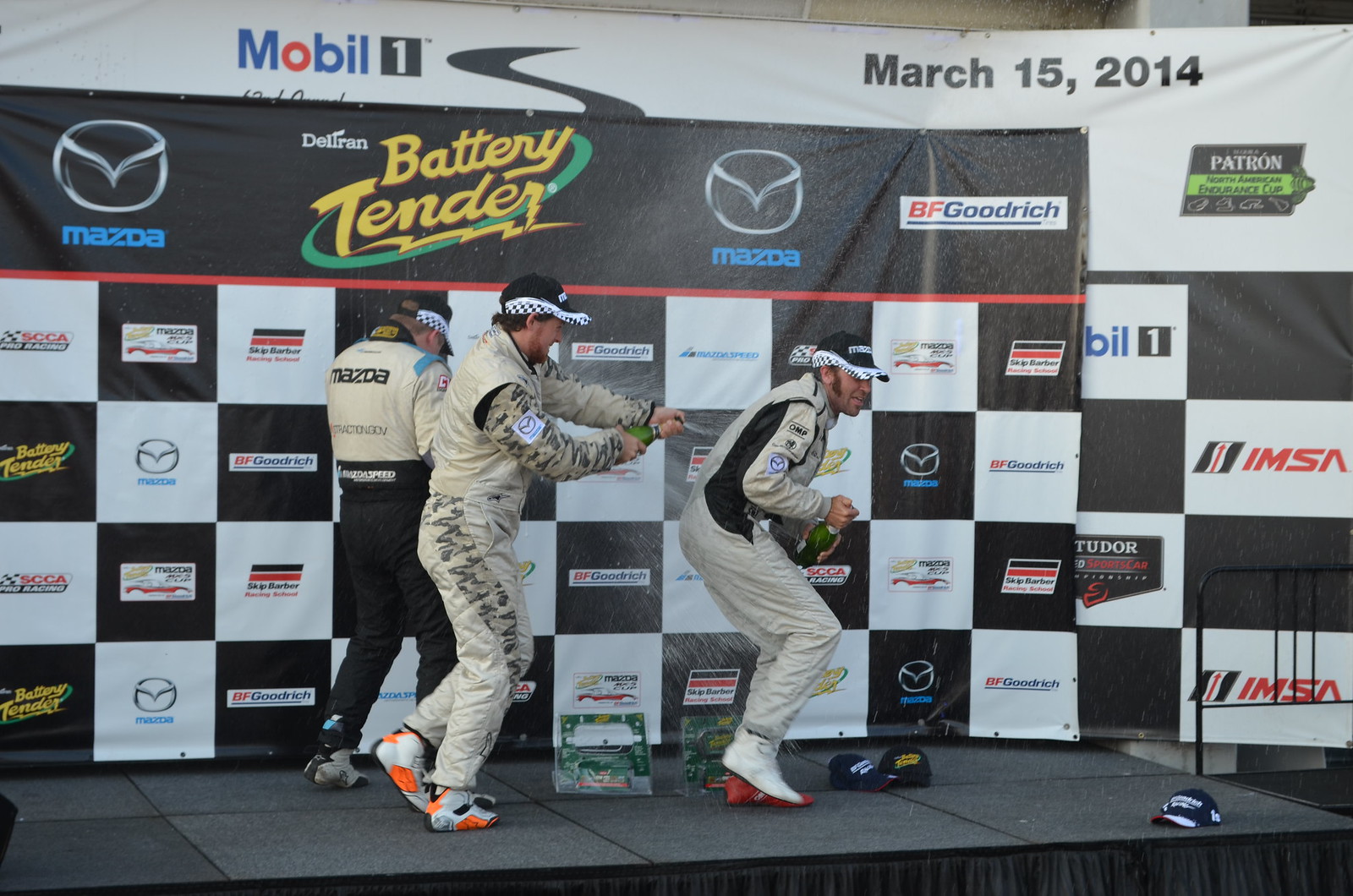The photograph captures an exuberant celebration on the Winner's podium after a road race, dated March 15, 2014. At the center of the image, two men dressed in tan racing uniforms adorned with the Mazda logo on their sleeves and checkerboard caps that also display the Mazda brand, are spraying champagne. The gentleman on the left directs the spray towards the man on the right, who is turning away to shield himself from the champagne. A third individual in the background is also turning away, retreating from the spray. The racing attire includes distinctive racing shoes and black-and-white garments, and the stage itself is black. Multiple sponsors such as BFGoodrich, Battery Tender, and Deltran are visible on the backdrop. The scene is vibrant with energy, capturing the triumphant moment shared among the racers.